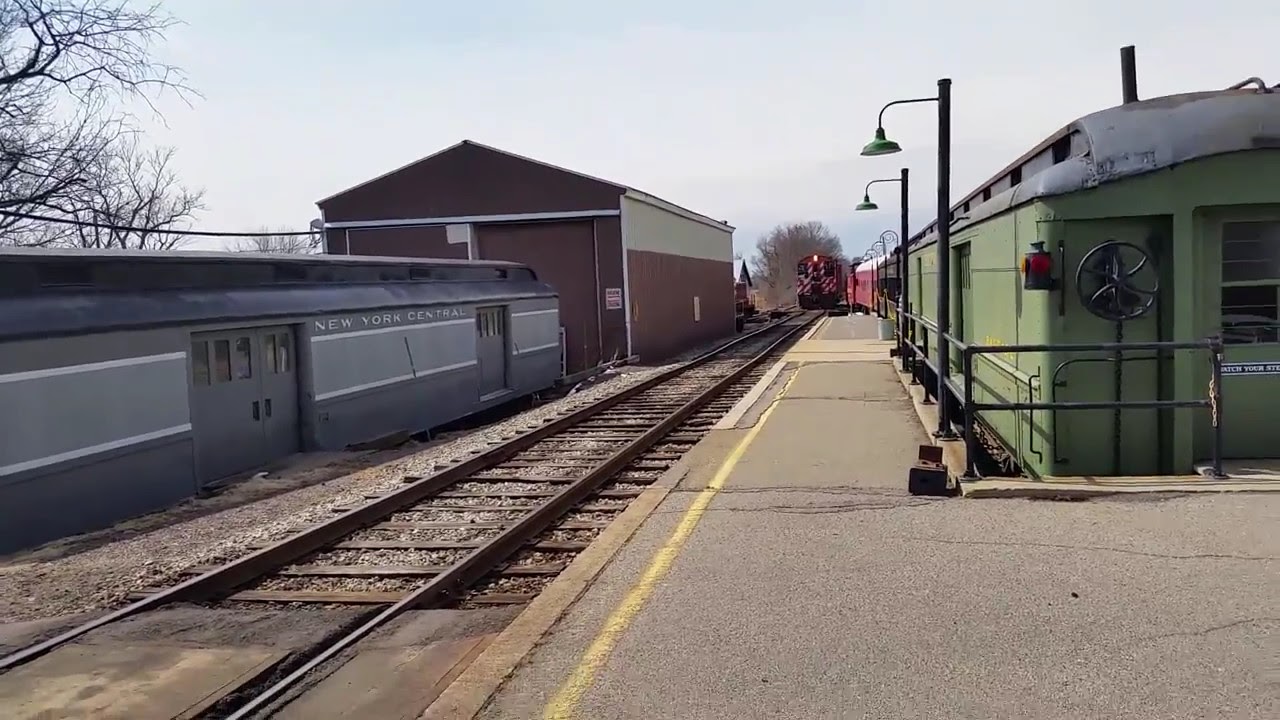The image captures a bustling outdoor train station. On the left-hand side, there's a prominent railway track beside which stands an old train with blue and gray stripes, marked with the words "New York Central." Adjacent to this vintage train is a brown metal building with a triangular green-topped roof, resembling a garage, where another train can dock. 

In the middle of the scene, a large red train with red and white stripes is seen approaching the station, its headlight glaring—a bright red light signals its arrival. The platform, devoid of people, is made of cement and features light posts, giving it a deserted charm. This central track area is flanked by trees in the background, with some cut-off branches visible, indicating the presence of greenery in this tranquil setting.

On the right-hand side, a recessed area houses another vintage train. This train is notably green with a black-painted roof and features an old doorway equipped with a metallic spinning wheel, alongside a classic train lantern with red and yellow lenses. In the background, you can spot a building resembling a storage warehouse with two large doors capable of accommodating a train. The overall weather is mostly clear with some clouds in the sky, casting a sunny yet slightly overcast ambiance over the quaint, vintage train station.